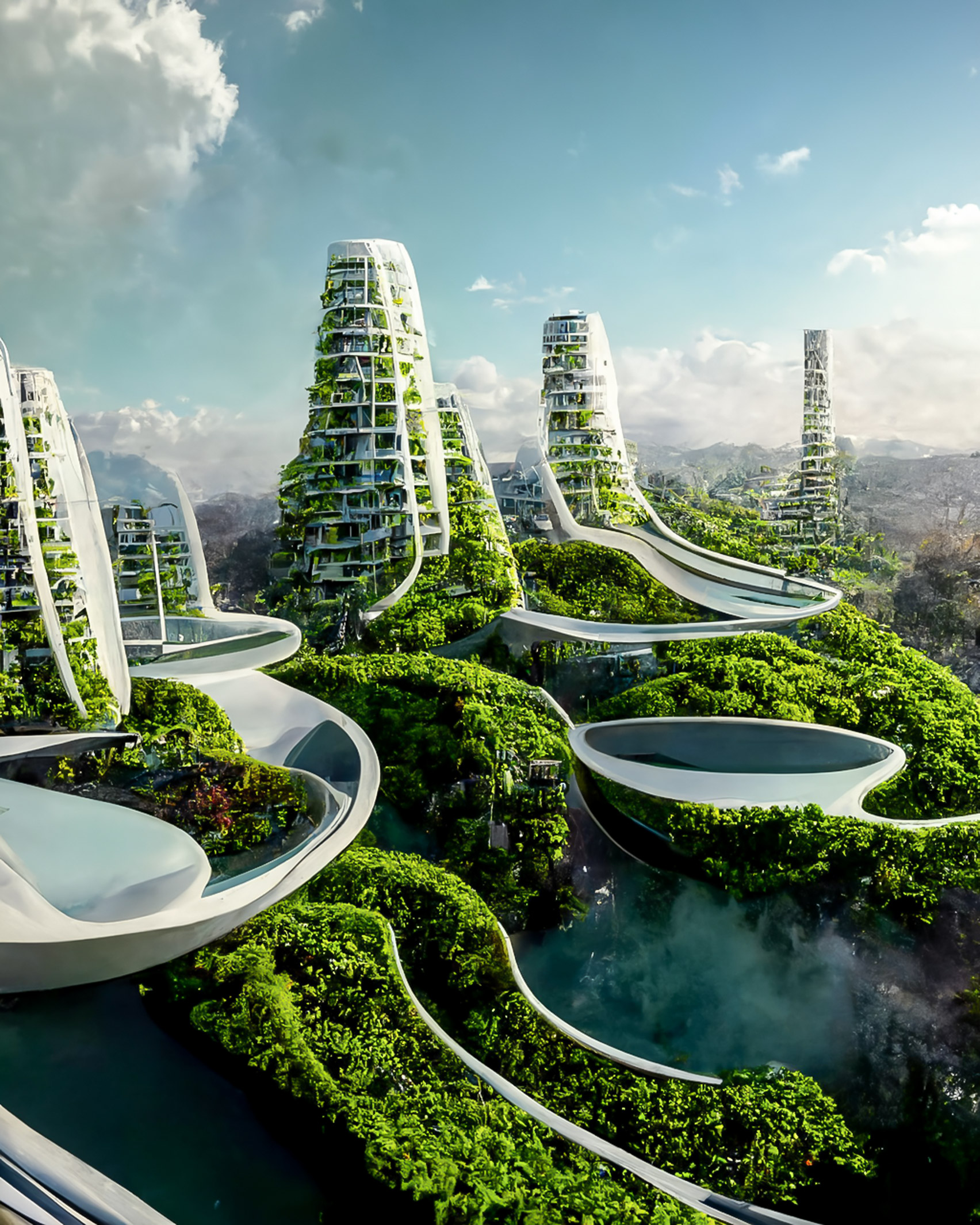The image showcases a stunning, AI-generated or digital representation of a futuristic cityscape set on a bright, sunny day with a blue sky adorned with clouds. The focal point is a group of towering, white buildings that merge modern architectural design with abundant greenery. These structures, potentially apartments or office buildings, are layered with several terraced levels and rounded bases. Each level features lush gardens and extensive plant life trailing down, integrating the buildings seamlessly with the surrounding verdant forest. Connecting these structures are numerous white pathways or slides, resembling water slides, which allow for pedestrian movement and other forms of transport. The entire scene appears to soar high into the sky, with a majestic view that reveals clouds and adds to the impression of an elevated, almost utopian environment. This visionary city harmonizes advanced urban living with nature, emphasizing sustainable and eco-friendly design.